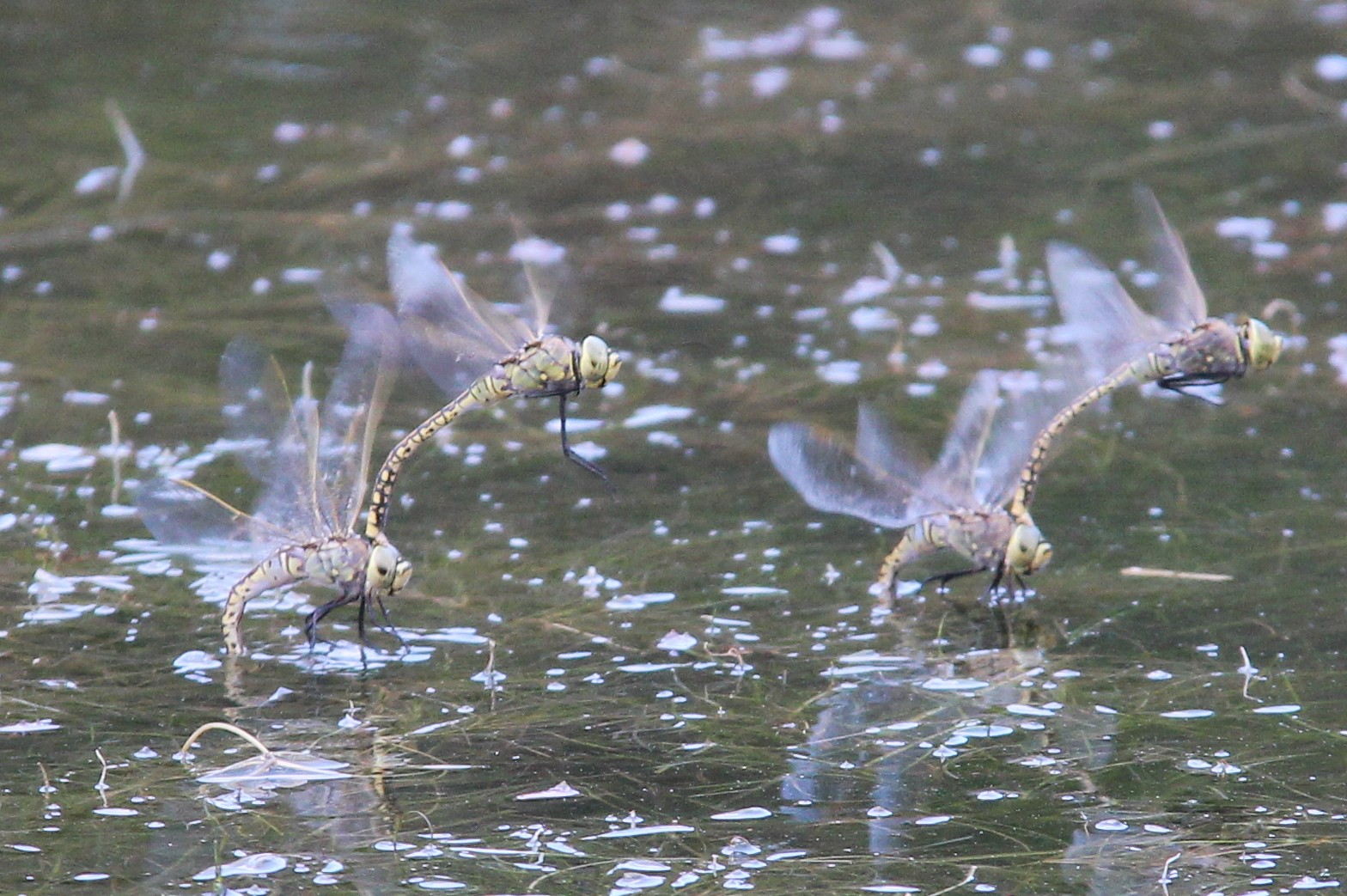In this captivating nature scene, the photograph captures a close-up of a tranquil, shallow pond, framed by delicate plant life and dotted with droplets indicating a light rain or recent sprinkle. The primary focus is on four dragonflies, their bluish-silver bodies and rapidly moving wings captured mid-motion. Arranged in pairs, two of the dragonflies are engaged in mating behavior, while the other two appear to be in various stages of emerging from the water. The blurred top half of the image, suffused with sunlight, adds a mystical aura, making the dragonflies' intricate wings shimmer against the watery backdrop. The clarity of the water reveals its shallow depth and the debris resting on the surface, enhancing the overall naturalistic charm of this serene pond scene.